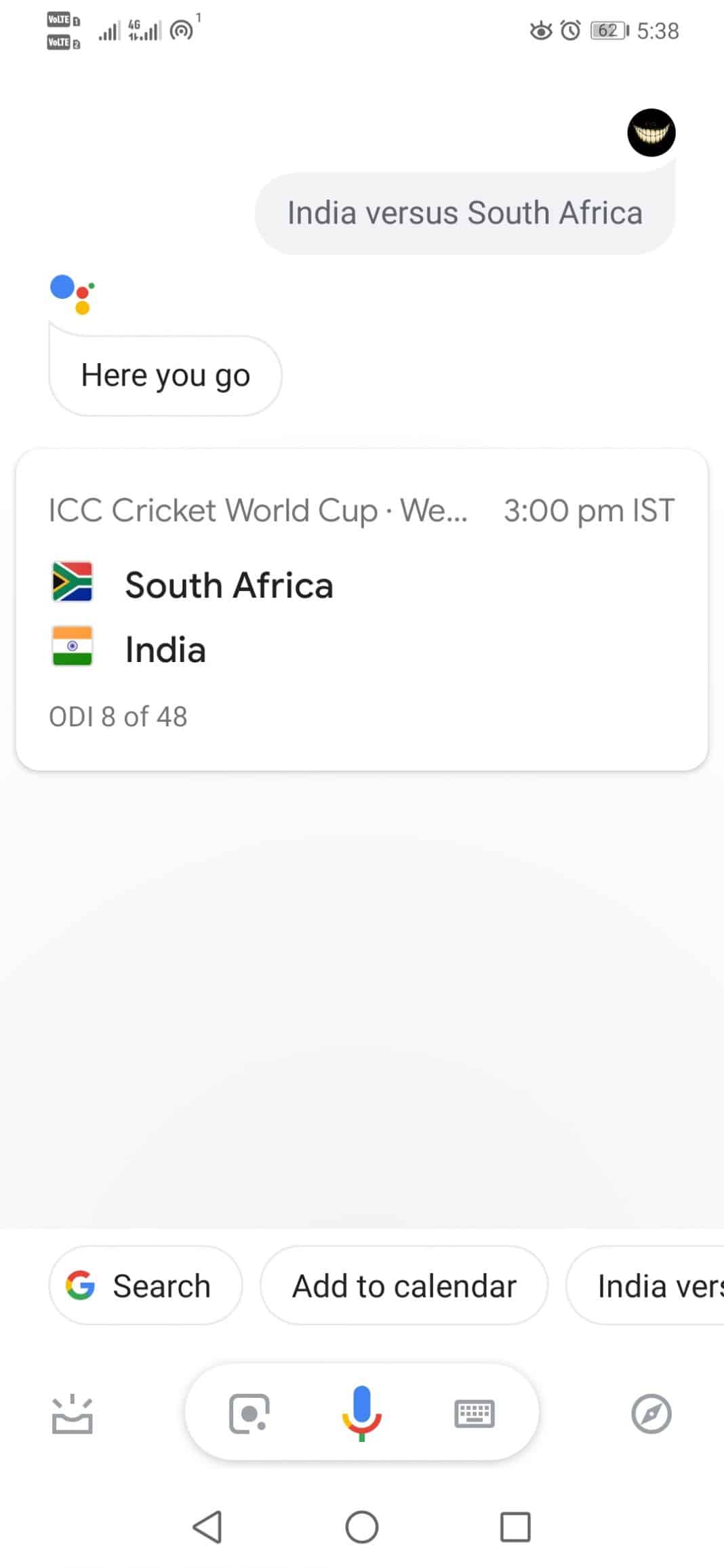A detailed and polished caption for the described image could be:

---

The screenshot depicts the results of a cricket match being viewed on a smartphone. In the upper left corner, the phone's signal bars are visible alongside notification icons. Notably, there is a stopwatch, an eye with eyelashes indicating 62% battery life, a clock showing the time as 5:38, and a user profile icon featuring a black circle with a Cheshire cat smile.

The main content on the screen highlights the ongoing ICC Cricket World Cup match between India and South Africa, with the event scheduled for 3 p.m. IST. The screen shows the South African and Indian flags next to the text "India versus South Africa." Additionally, the Google Assistant icon on the left side of the panel displays the phrase "Here you go."

The match details are displayed on a floating white panel with a very subtle outline. Below the primary information, there is substantial white space. The footer of the panel reads "G search at the calendar India VRS," although it is cut off. 

Below this floating panel, the screen features several operational icons: an inbox icon, a photo or camera icon, a colorful microphone icon, which contrasts the otherwise grayscale icons for the keyboard and navigation compass. At the very bottom, a standard navigation menu is presented in grayscale.

The rest of the screen maintains a minimalist aesthetic with simple grey and black text on a white background.

---